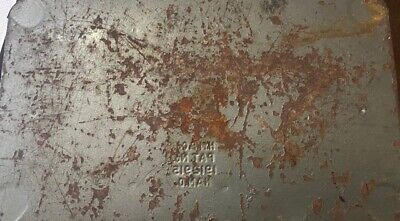This is a highly detailed close-up photograph of a large piece of old, corroded metal occupying almost the entire frame, except for a small section in the upper left-hand corner where a jagged, ragged edge is visible against a light background. The metal is dull, medium gray with extensive rust patches that range from large, globular orange-red-brown spots mainly in the center to smaller specks and lines along the edges, giving it a heavily damaged and worn appearance. The metal surface is also marred by numerous scratches and etched lines.

In the bottom center of the metal, there is a stamped, backward inscription that appears to include a patent number, obscured by rust and corrosion, making it difficult to read completely. The letters are imprinted in the metal in such a way that they would be more legible in a mirror image. The inscription might contain Cyrillic characters, suggesting it could be something historical, possibly a piece of ammunition from World War II, although its exact origin is unclear due to the extreme close-up nature of the photo. The main focus of the image is the texture and degradation of the metal, emphasizing the rust and wear over time.